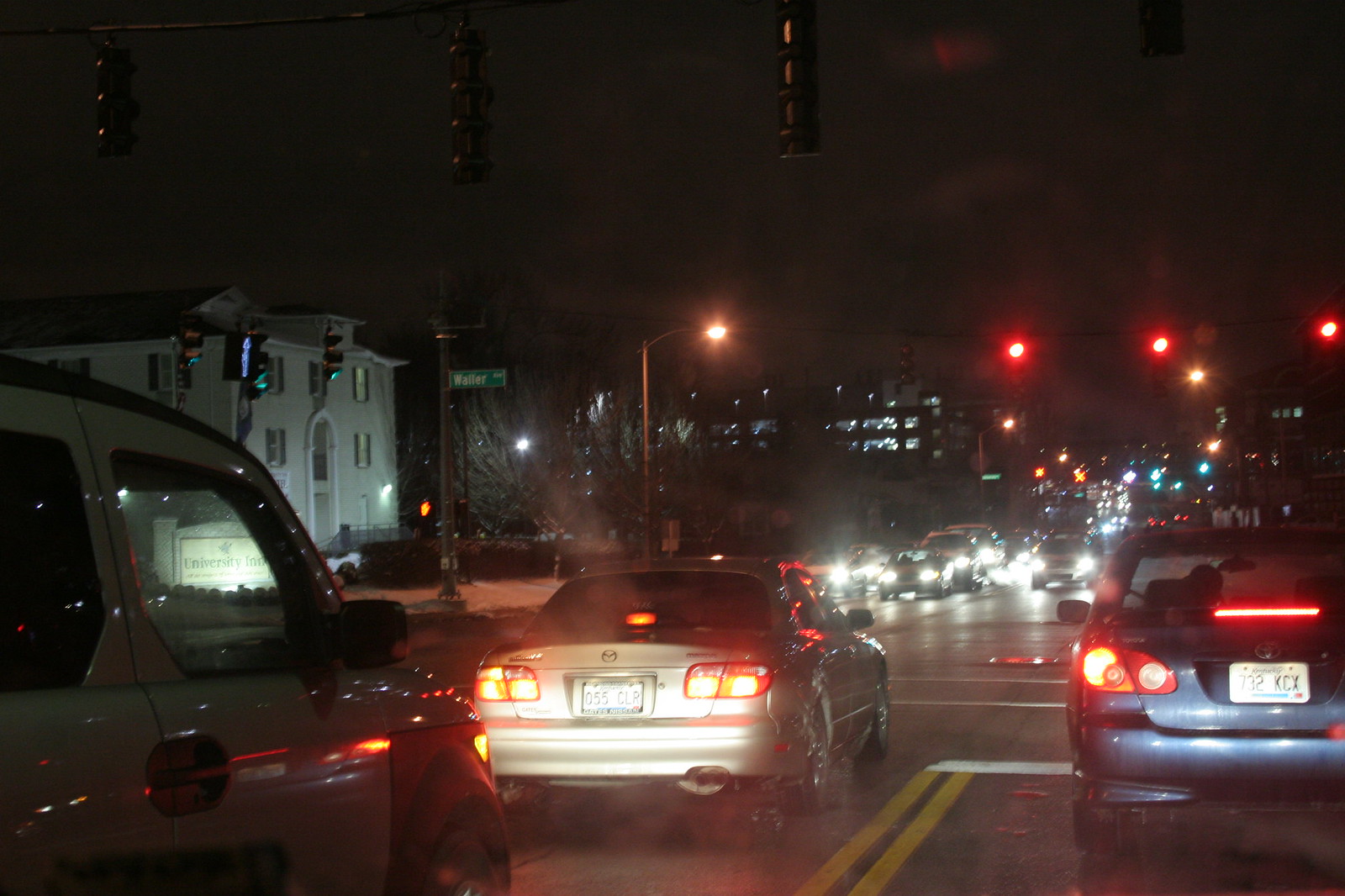In this nighttime photograph taken at an intersection, the traffic light shines red from the perspective of the camera. Dominating the left-hand side foreground of the image is a white, boxy car with an orange front. Directly ahead of this vehicle is a silver Toyota Corolla, with a blue Toyota Corolla positioned to its right. The scene is teeming with oncoming traffic, as headlights stretch into the distance, illuminating the road far into the horizon. On the left side of the frame, a three-story, square brick building stands prominently against the dark sky.